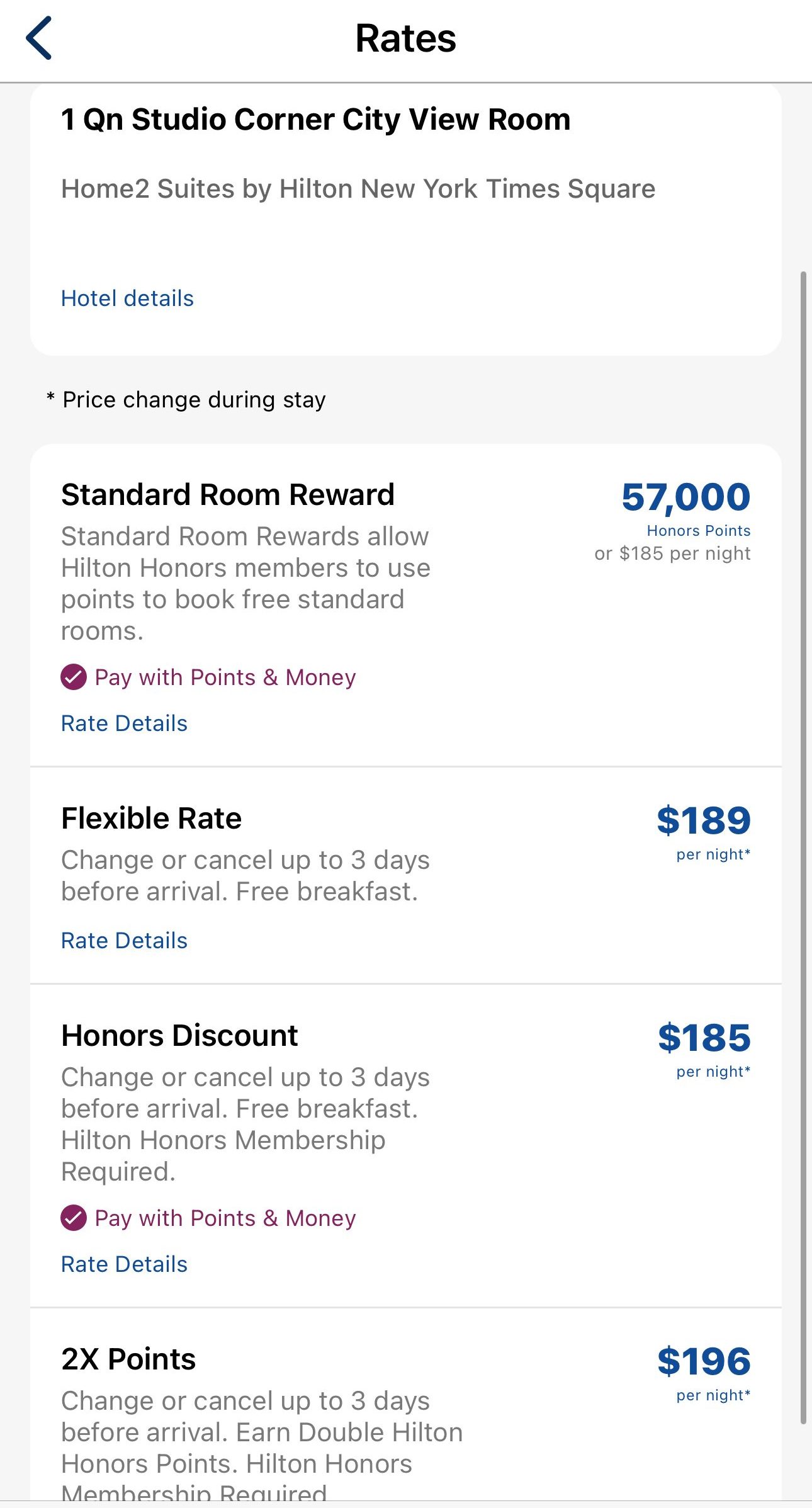The vertical rectangular image features a light gray background adorned with multiple white boxes. At the very top of the screen, "Rates" is prominently displayed in black text, accompanied by a back arrow on the left. Directly below this, more black text announces "One QN Studio Corner City View Room," with the subheading "Home2 Suites by Hilton New York Times Square" in gray text. This information is enclosed within a clean white rectangle.

Moving down the image, the phrase "Price change during stay*" is written in black on the gray background. Following this, another white box appears with "Standard Room Reward" at the top in black text. Beneath it, gray text explains that "Standard Room Rewards allow Hilton Honors members to use points to book free standard rooms." On the right side, bright blue text displays "57,000 Honors Points or $185 per night."

Lower in this box, bright purple text invites users to "Pay with Points and Money," accompanied by a purple circle containing a white checkmark. Below this, "Rate Details" is highlighted in blue.

The final white box is titled "Flexible Rate" in black text. Underneath, gray text provides further details: "Change or cancel up to three days before arrival, free breakfast." This option is listed at "$189 per night."